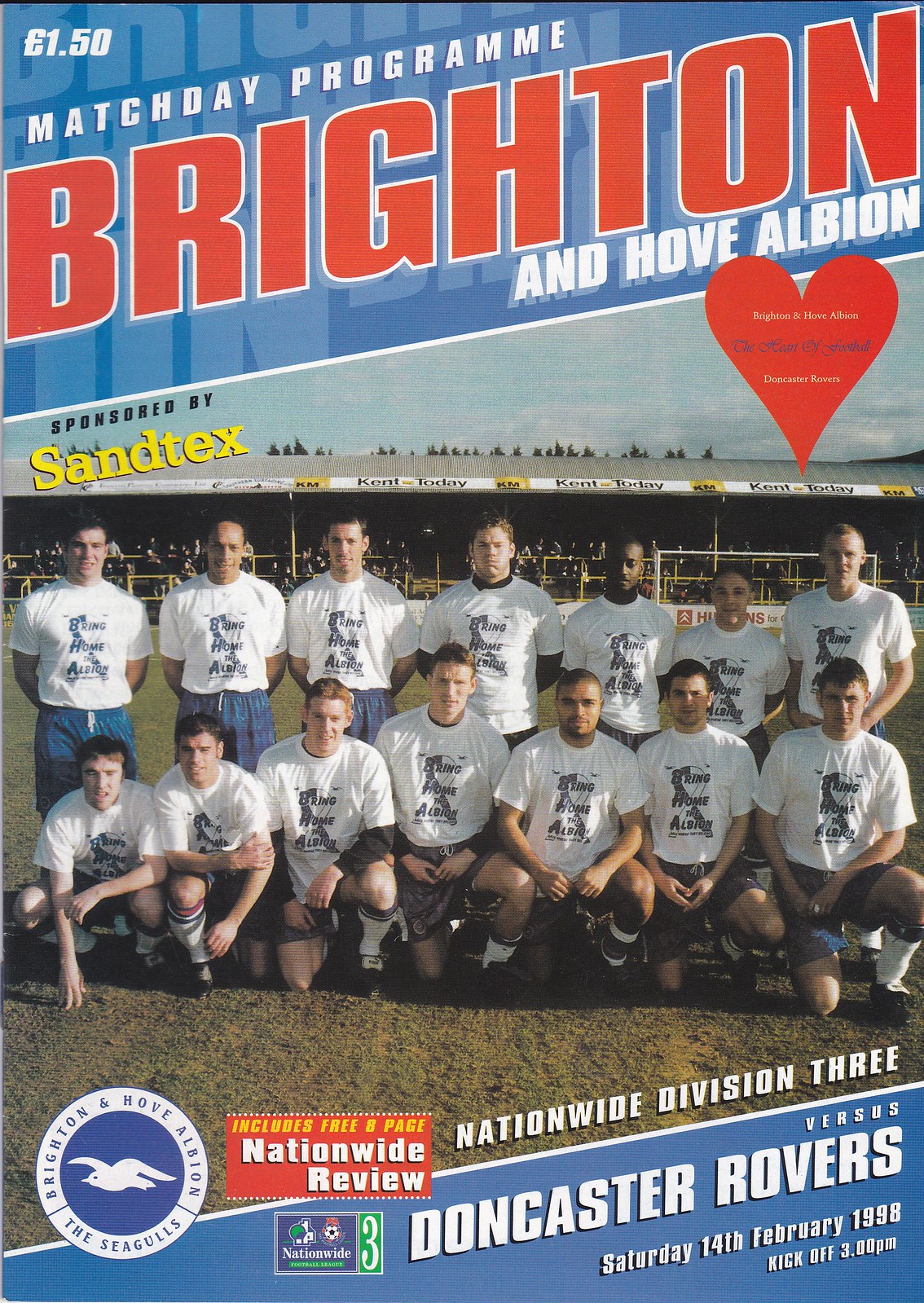The cover of this colorful Match Day Program for a soccer game features a vibrant mix of red, white, and blue. Dominating the center is a photograph of the Brighton and Hove Albion team, positioned on a grass field with spectators visible in the background. The team is arranged in two rows: the front row kneels while the back row stands, all donning white shirts and blue shorts emblazoned with the slogan "Bring Home the Albion."

Across the top left corner in white text, the price is displayed as "1 pound 50." Below that, in the same color, it reads "Match Day Program." The program's title is highlighted in bold red letters with a white border stating "Brighton," and beneath it in white text, "An Hove Albion." The cover notes sponsorship by "Sandtex" in black and yellow text at the upper left quadrant.

At the very bottom right of the cover, the details of the match are given: "Nationwide Division 3 versus Doncaster Rovers, Saturday 14th, February 1998, kickoff 3pm." Additionally, a red box promises an "Includes Free 8-Page Nationwide Review," next to a Nationwide branding logo. A distinctive circle logo bearing the text "Brighton An Hove Albion, the Seagulls," with a seagull illustration, is also positioned towards the bottom.